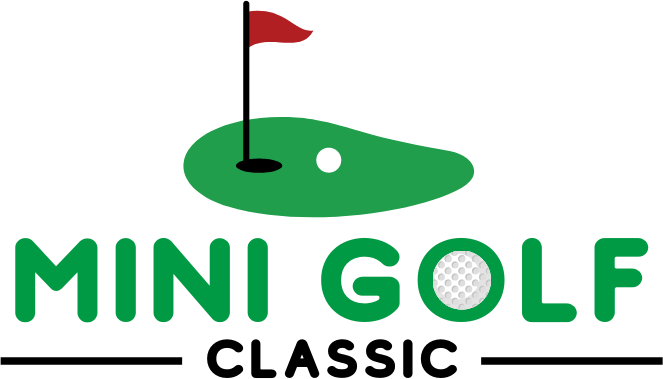The image is a computer-generated logo for a video game titled "Mini Golf Classic," reminiscent of older Nintendo games. The text "MINI GOLF" is prominently displayed in large, green, all-caps letters, with a unique design: the "O" in "GOLF" is a golf ball encircled by the letter. Below this, "CLASSIC" is written in black capital letters, flanked on both sides by partial horizontal lines that connect to the underlining of "MINI" and "GOLF." Above the text, there's a detailed graphic of a putting green featuring a red flag atop a black pole, inserted into a black hole. In front of the hole rests a white golf ball. The flag is depicted as a slightly wavy red triangle. The entire logo is set against a transparent white background, creating a cohesive and visually appealing design.